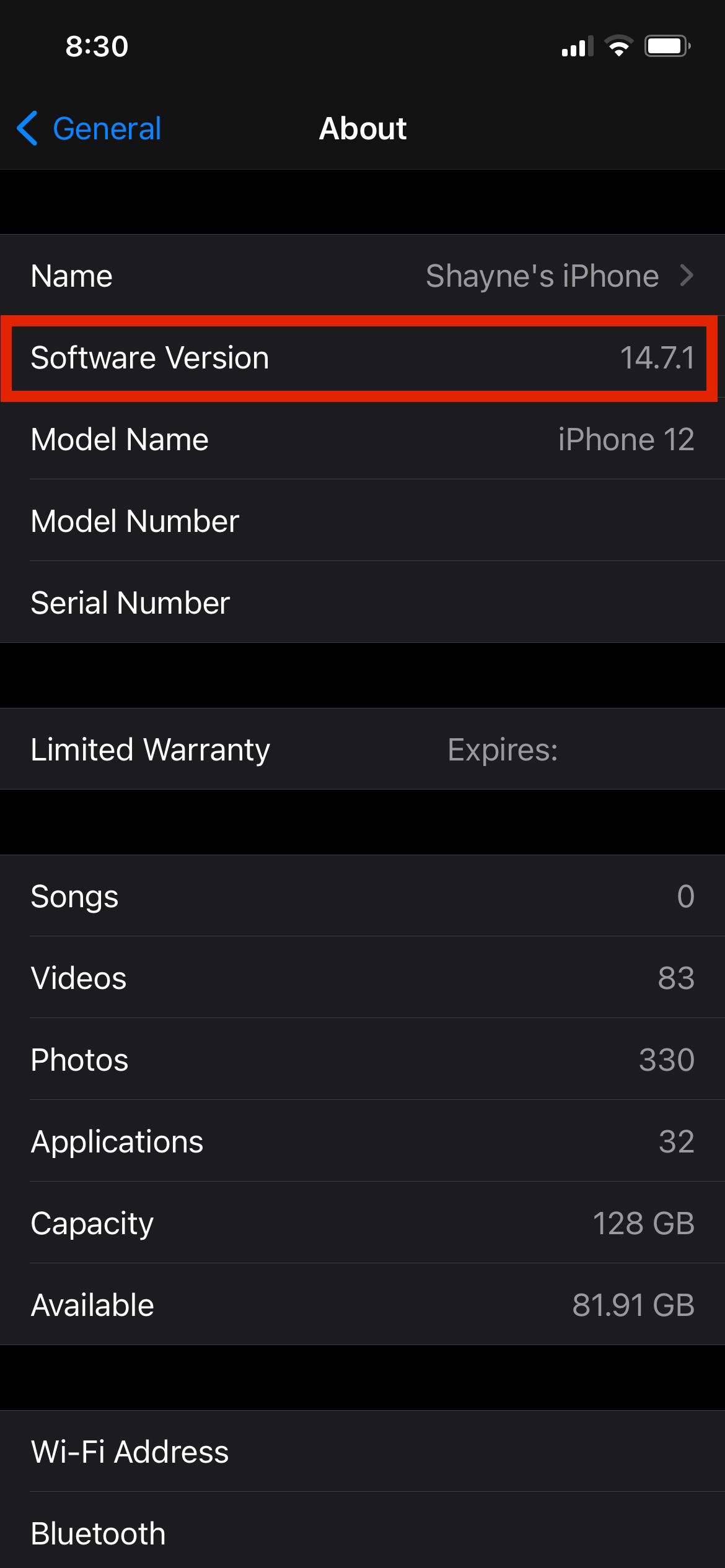A screenshot of an iPhone's settings page is captured in this image, showcasing detailed device information. In the top right corner of the screen, the battery icon appears almost full, likely indicating a charge of over 90 percent. To the left of this, the WiFi icon displays 2 out of 3 bars, and the phone signal strength icon shows 3 out of 4 bars. On the top left, the screenshot capture time is noted as 8:30. Centrally positioned at the top, the text "About" in white is visible, with "General" and a left-pointing blue arrow situated to its left.

Immediately below, the first section displays device-specific details: "Name" listed as "Shane's iPhone" on the right, followed by "Software Version 14.7.1", both enclosed in a red rectangular border. Subsequent entries include "Model Name" set as "iPhone 12", "Model Number", and an unspecified "Serial Number".

In the next section, the "Limited Warranty" is mentioned, indicating it is expired without specifying a date. 

Detailed storage and media information follows in the concluding section: "Songs" counted at 0, "Videos" at 83, "Photos" at 330, and "Applications" totaling 32. The device capacity is 128 GB with 81.91 GB available. The lower-most part of the image references "WiFi Address" and "Bluetooth".